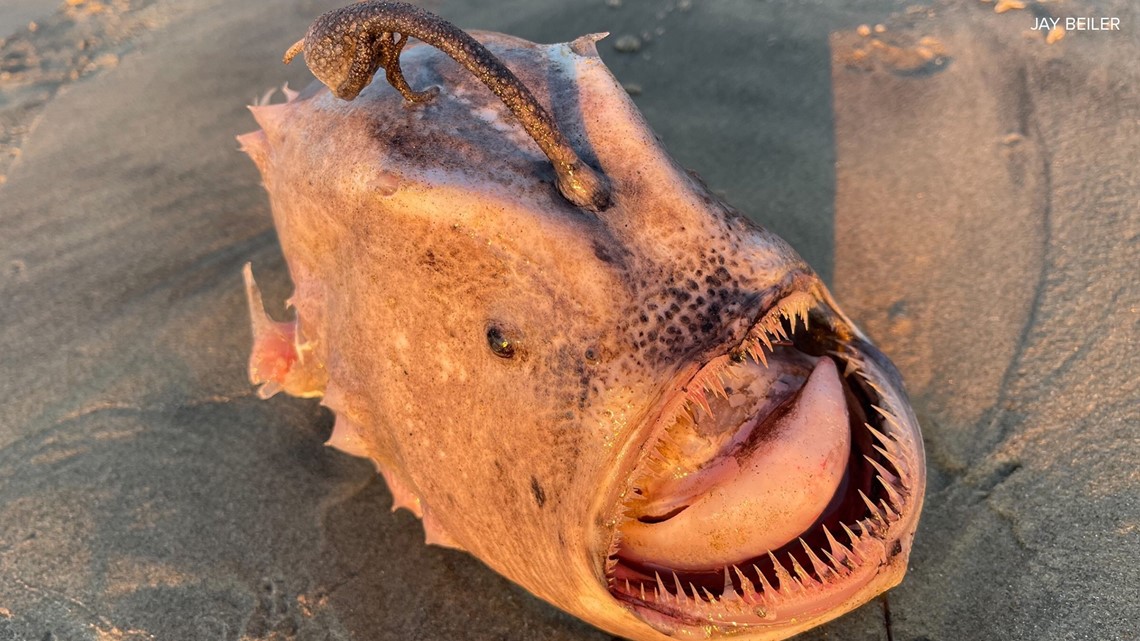In this striking photograph, a large, partially petrified sea creature is starkly displayed on a moist, medium-brown sandy shore. The creature prominently features a massive light brown head with a menacingly wide-open mouth, revealing numerous narrow, jagged teeth. A particularly massive tongue is visible, protruding slightly from the gaping maw. Adding to its intimidating appearance, a dark gray, horn-like structure emerges from the top of its head, curving around in a hook-like shape. Speckled black spots are noticeable just above its top lip. Captured primarily from the right side and slightly angled downward, the photo also highlights one of the creature’s side eyes, accentuating its daunting presence. As a final detail, small white text in the upper right-hand corner reads the name "J. Beiler," reinforcing the image's authenticity.